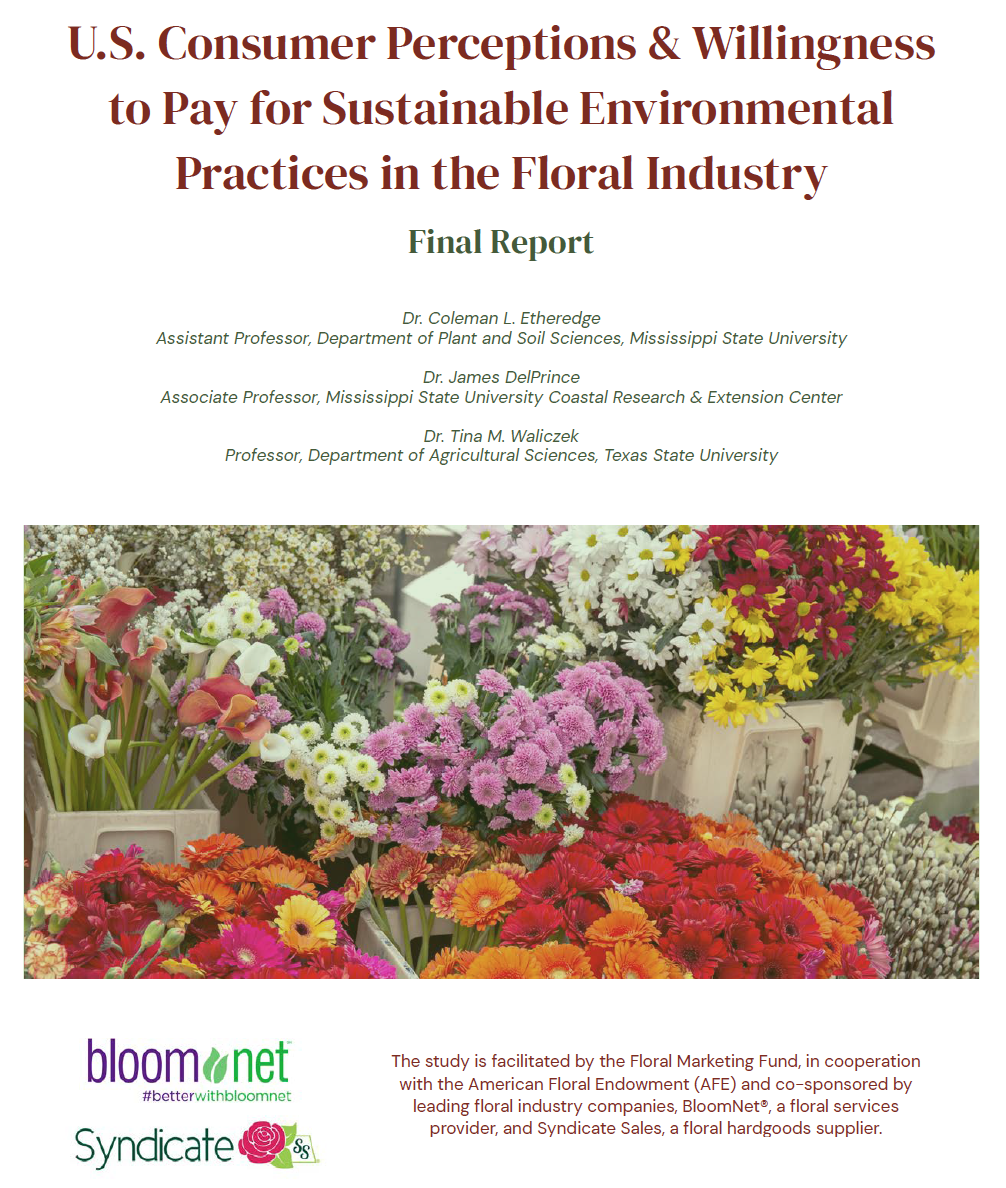The image is a detailed advertisement featuring text and a vibrant photograph. At the top, written in red text, is the title: "U.S. Consumer Perceptions and Willingness to Pay for Sustainable Environmental Practices in the Floral Industry." Below, in green text, it states: "Final Report." The names of the contributing professors are listed as Dr. Coleman L. Etheridge, Dr. James Del Prince, and Dr. Tina M. Walaszczyk, with their respective affiliations. Beneath the text is a colorful and dynamic photograph of diverse floral arrangements, showcasing flowers in pink, yellow, red, purple, orange, and white, in various sizes and shapes. The bottom of the image features the logos and names of BloomNet, with a green rose logo, and Syndicate, with a red rose logo. Additionally, it mentions the study being facilitated by the Floral Marketing Fund in cooperation with the American Floral Endowment (AFE) and co-sponsored by leading floral industry companies, BloomNet and Syndicate Sales.